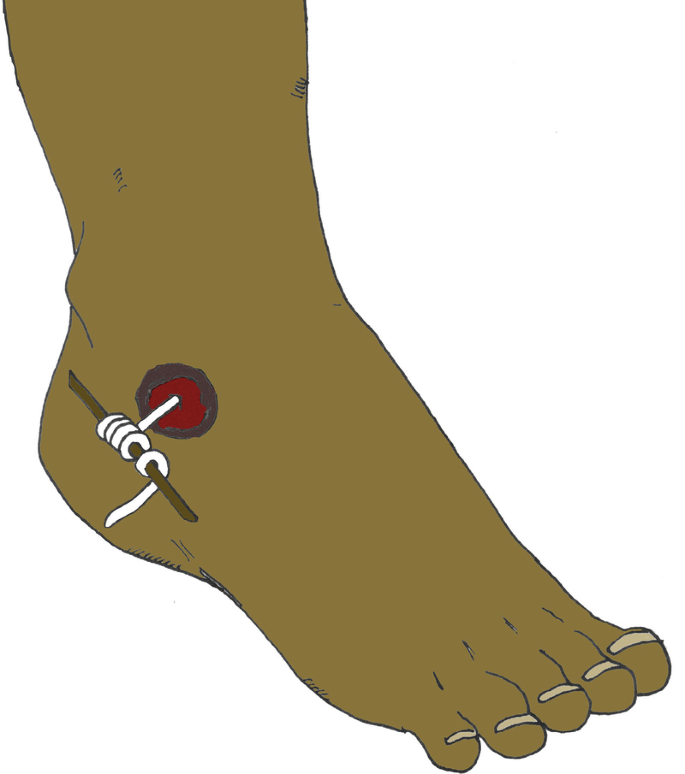The illustration depicts a right foot with dark skin, seen from just above the ankle down to the toes, set against a solid white background. Located just forward of the ankle and above the heel, a circular wound with blackened edges reveals a bright red interior, indicating the presence of blood. Emerging from this wound is a thin white wire or tube, which is coiled around a small brown stick positioned parallel to the foot. The exact nature of the object being pulled from the wound is unclear, but its appearance resembles a worm wrapped around a stick. Overall, apart from the wound, the foot itself is unremarkable.